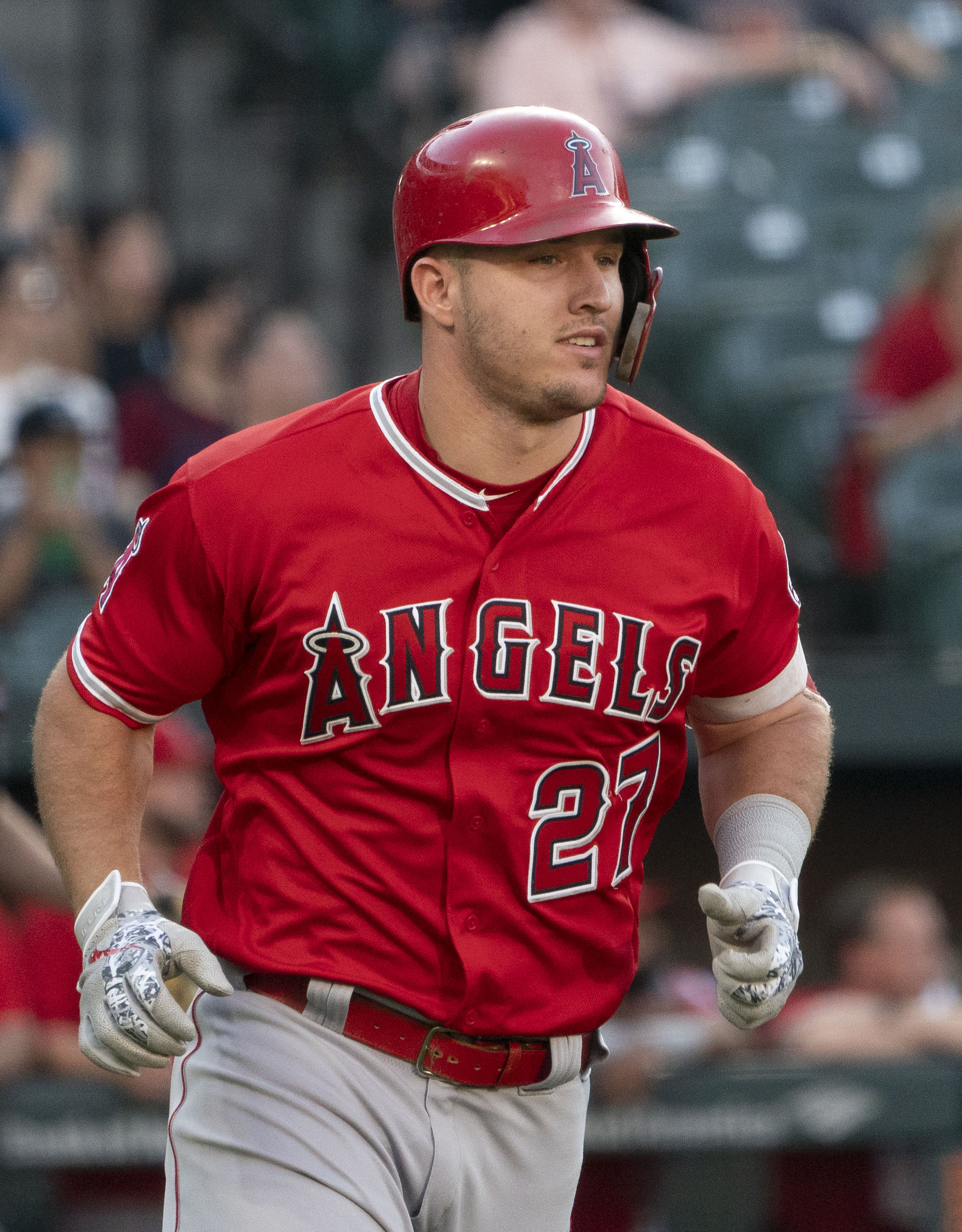The image features Mike Trout, a prominent baseball player for the Anaheim Angels, captured in mid-run. He is donning the red and white Angels uniform, with the number 27 emblazoned on his jersey. Across the front of his red jersey, the word "Angels" is displayed, with the distinctive red "A" sporting a white halo. His outfit includes white batting gloves, a red belt, and white pants. Mike Trout is also wearing a red batting helmet, similarly adorned with the Angels' logo. He has a bit of scruff on his face, visible under the helmet. The background of the photograph shows a blurry view of the stands filled with spectators, emphasizing the action and focus on Trout. The natural daylight suggests that the game is taking place during daytime. The overall scene captures the dynamism of Trout likely after making a significant play, such as hitting a home run, given his poised yet active stance.